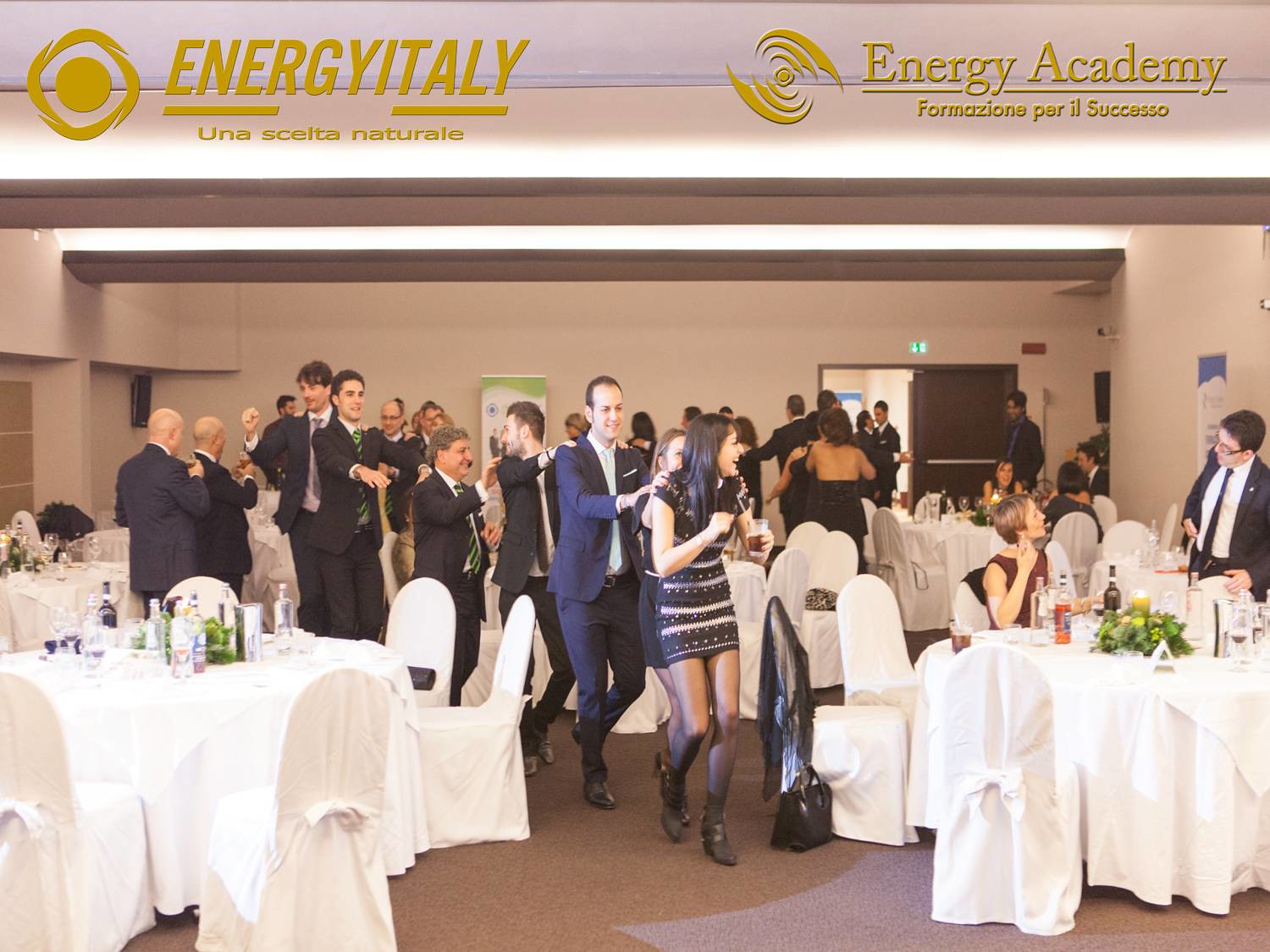The image captures a lively indoor gathering in a ballroom, seemingly an office or corporate event. The room features tables adorned with white tablecloths and matching white tie-back chairs. Beige walls and drop-ceiling lighting set the ambiance. Prominent at the top of the image are the phrases, "Energy Italy, Una Escleta Natural," and "Energy Academy, Formacion por el Sacaso," written in yellow against a pink background, with their respective logos beside them. In the upper right corner, an emergency exit sign hangs above a double brown door, with people visible in the doorway.

A conga line snakes through the room, led by a woman in a short, almost sleeveless dress featuring black, white, and brown patterns. Following her, several men dressed in suits join in the dance, adding to the festive atmosphere. There are also a few women in cocktail dresses scattered in the crowd. On the lower right, a woman seated at a table engages in conversation with a man standing next to her. The setting, complete with circular tables and a mix of dancing and seated guests, exudes the vibrant and celebratory spirit of the event.